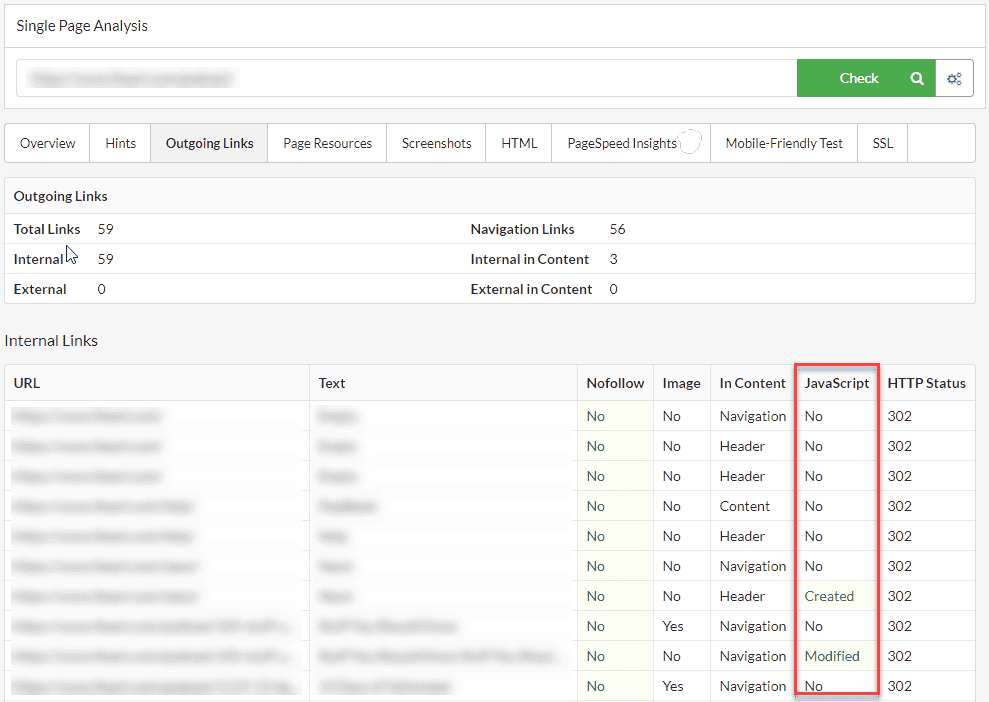In the image of the website, a detailed interface layout is displayed. At the top, a long black banner with the title "Single Page Analysis" is prominently featured. Below this banner is a search bar, although the text within this bar is intentionally blurred out. Adjacent to the search bar, there is a vibrant green button labeled "CHECK" in capitalized white text, accompanied by a white magnifying glass icon. 

Scrolling further down, the navigation options include "Overview," "Hints," "Outgoing Links," with "Outgoing Links" highlighted by a gray background. Additional menu options listed are "Page Resources," "Screenshots," "HTML," "Page Speed Insights," "Mobile Friendly Test," and "SSL."

The section under "Outgoing Links" provides detailed metrics, displaying various link categories including "Total Links," "Internal Links," "External Links," "Navigation Links," "Internal in Content," and "External in Content." 

In the "Internal Links" section, the details span several categories: "URL," "Text," "Nofollow," "Image," "In Content," "JavaScript," and "HTTP." Notably, the "JavaScript" category is highlighted with a red perimeter. The subsequent entries under each category list repeated "No" indications, except for "Created" and "Modified," which also say "No." However, all URLs and texts within this section are blurred out, ensuring sensitive data remains obscured.